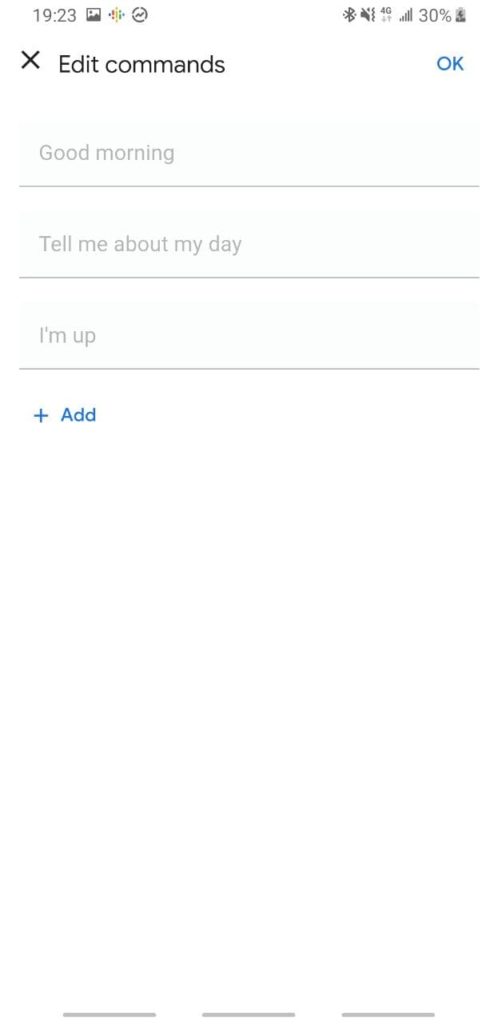This image, captured on a smartphone, depicts a screen with several interface elements. At the top of the image, there is an edit command section, featuring a prominent black "X" on the left side for closing or canceling actions, and on the right side, the word "OK" displayed in teal. Below these options, the phrase "Good morning" appears in gray text, positioned above a faint gray line that stretches horizontally across the screen.

Further down, the text "Tell me about my day" is shown, followed by another faint gray line. Beneath this, the words "I'm up" are displayed, with yet another faint gray line below them. Underneath this section, in blue text, is a "+" symbol accompanied by "Add" (capital 'A' followed by lowercase 'd's).

The bottom portion of the image is largely plain white, except for the very bottom edge, which features three short, dashed gray lines. These lines are evenly spaced, alternating between gray and clear segments.

This screen capture appears to show a morning routine or daily planning interface, with various prompts and options for user interaction.